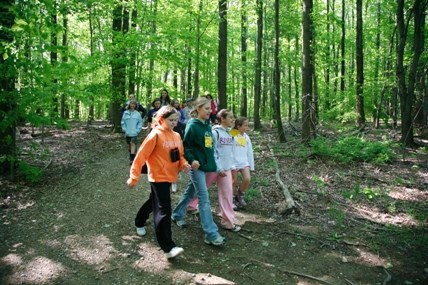In this small, horizontal, rectangular image, a scene unfolds in a sunlit park or wooded area, where a group appears to be enjoying a nature hike. Dominating the foreground is a trio that could be a family unit, possibly a mother and her two daughters, all appearing to be female. The child on the left wears an orange sweatshirt and black pants, slightly taller than her sister on the right, who sports pink pants and a white shirt. The mother, identified by her height and mid-position, is clad in a green sweatshirt and blue jeans. All three seem to be walking on a well-trodden dirt path surrounded by trees with lush green foliage. Ahead, the sunlight dapples the ground, adding a warm glow to their surroundings.

In the background, another family group, partially obscured, includes at least one adult and one child, hinting at the possibility of more individuals hidden from view. The setting suggests a frequent-use path through the woods, evidenced by the bare, vegetation-free ground underfoot. The overall impression is that of a serene, shared moment amidst nature, possibly part of a school-organized outing or a communal family hike, capturing the essence of togetherness and the joy of outdoor exploration.